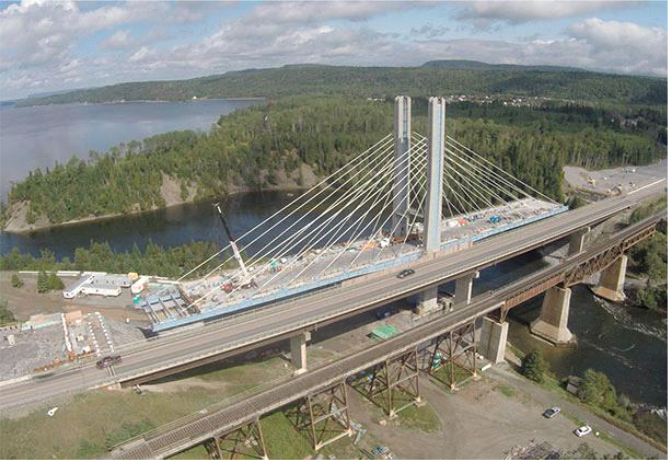This aerial, horizontally aligned rectangular photo captures a striking scene combining elements of sky, land, water, and a prominent bridge. At the top of the image, the blue sky is dotted with numerous puffy white and gray clouds. Just beneath the sky, there is an expanse of hilly, green land that stretches across the background. Towards the upper left section of the photograph, a calm, grayish body of water—resembling a lake—can be observed. Cutting across the landscape horizontally, a strip of land adorned with tall trees traverses from left to right.

Midway down the image, another body of water appears, this time with a brownish hue. The most striking feature is the large bridge that spans diagonally from the lower left to the upper right. This bridge is supported by two main structures featuring wires descending in an upside-down V shape at each end. The bridge appears to be mirrored by another bridge below it, which might be under construction as no cars are visible on either structure. 

Adjacent to the bridge, a highway runs parallel, possibly indicating that the older bridge is no longer in use or is undergoing repair. Notably, the right end of the bridge looks broken off, suggesting disrepair or planned demolition. Below the highway is a dark, possibly paved area that could be a walkway, and further down, the ground appears to be a mix of brown and green hues. This area features some greenery and in the distant background, the hilly, tree-covered landscape extends, framing the bridge and leading back to the water to the left. This intricate layering of natural and man-made elements provides a vivid snapshot of an evolving landscape.